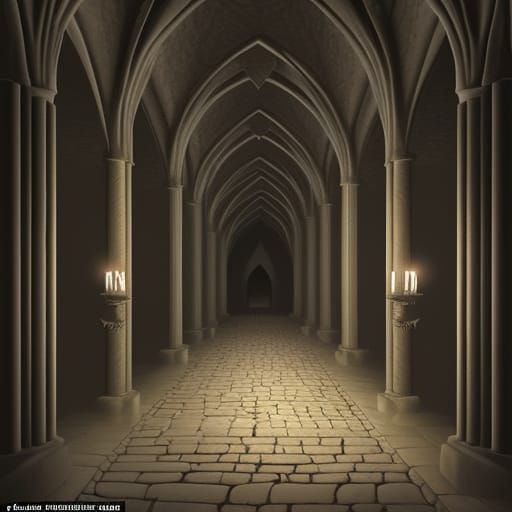This digital illustration depicts the interior of a dimly-lit, castle-like hallway rendered in shades of brown, black, and gray. The hallway extends back to a dark, arch-shaped doorway, with its pointed top mirroring the arches along the walls. These arches rest on light brown columns that line both sides of the corridor, twelve in total, and ascend towards a beige-toned ceiling. The cobblestone floor, littered with visible cracks, is a light brown shade. The dim illumination is provided by lit lanterns and tall white candles positioned in sconces on the pillars, casting light in the otherwise shadowy passage. The walls themselves are dark, almost black, enhancing the gothic and eerie atmosphere of the scene. At the bottom left of the image, there is a small, unclear text within a black rectangle. Overall, the scene evokes a strong sense of fantasy and mystery, reminiscent of ancient castle hallways.